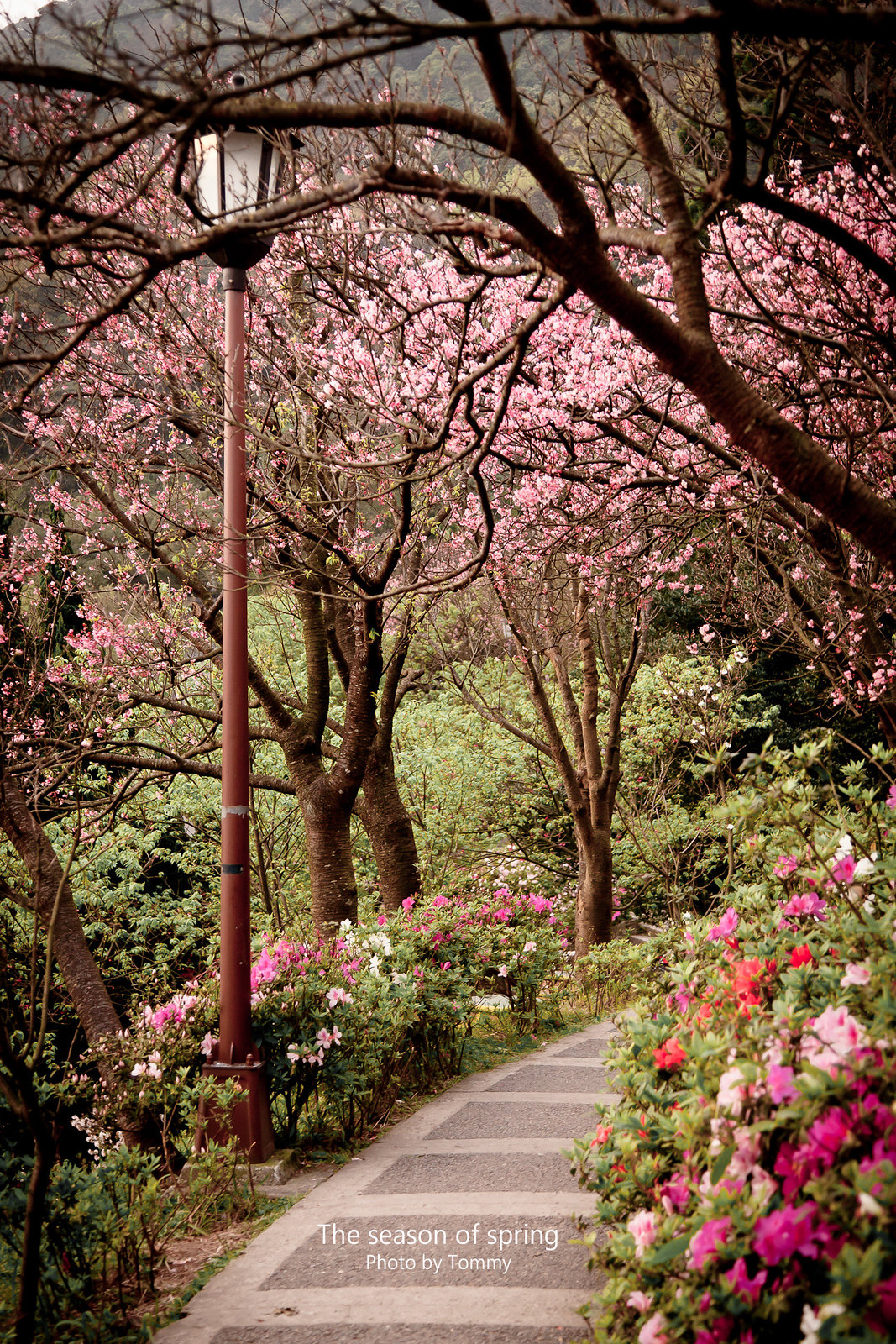In this vivid photograph of a beautiful garden, a cement footpath or walkway cuts through the scene, lined on both sides with colorful flower bushes featuring roses and carnations in shades of pink, red, and purple. Towering above the blooms are large trees adorned with delicate, pastel cherry blossoms in shades of white and pink. To the left of the walkway, a tall, vintage-style lamppost, reminiscent of the 1950s and constructed from black metal with glass panes, stands elegantly, though its light is not illuminated in the daytime setting. Alongside the path, the left side dips into an embankment dense with lush greenery and additional bushes, adding to the garden's enchanting atmosphere. The top of the image is overlaid with white text that reads "Spring, photo by Tommy." The overall scene exudes a tranquil, springtime charm.